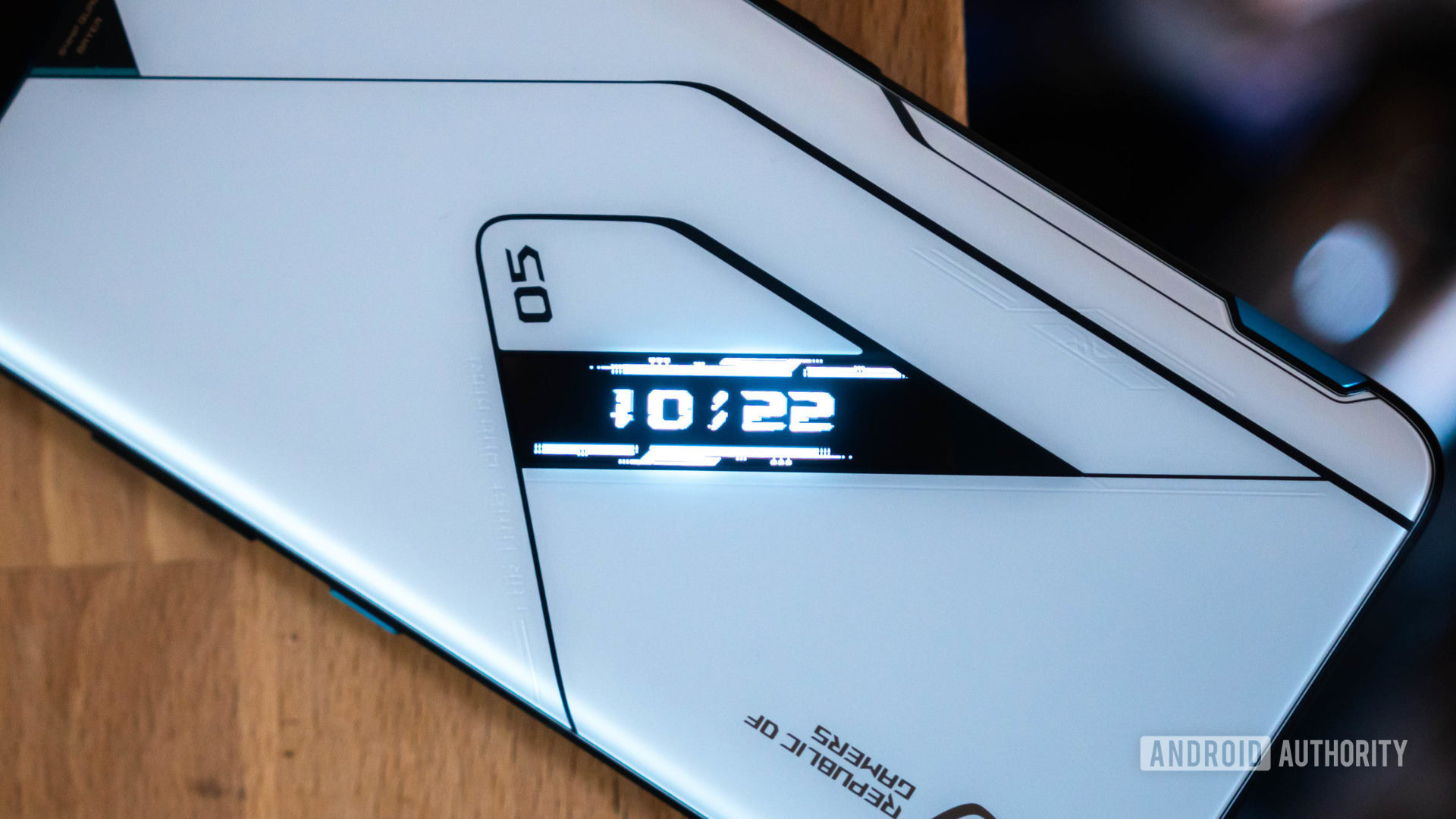The image showcases a futuristic gaming console, prominently positioned diagonally from the top left to the bottom right. The console, which features a sleek design in silver and white with geometric black lines and a blue button on its side, displays the text "10-22-05" in the center and "Republic of Gamers" below it. The device rests on a light brown wooden table, occupying the left two-thirds of the image. The background on the right third is blurred with dark indigo or black tones. Additionally, in the bottom right corner, there is white text stating "Android Authority" on the black background. The overall style of the image suggests a high-end, on-display presentation typical of advanced gaming technology.